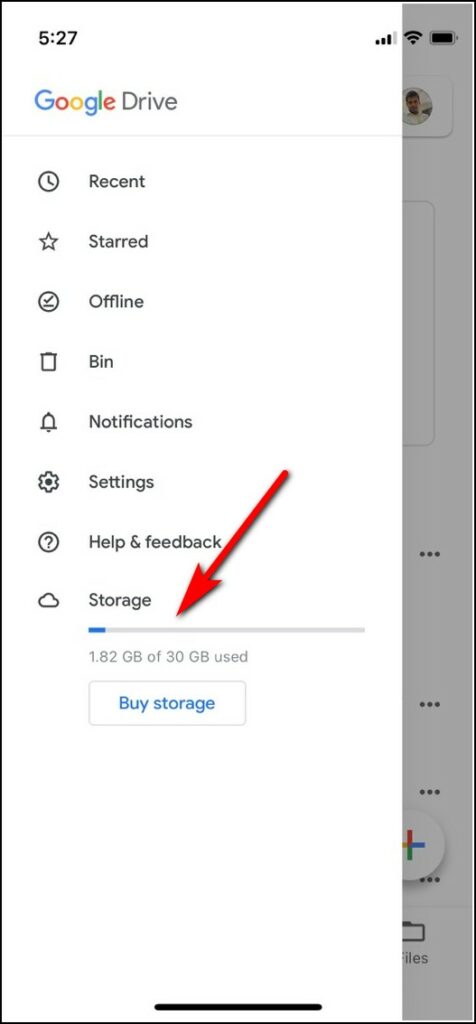Image Caption: 

A close-up of a smartphone screen displaying an open Google Drive app. The time on the device is 5:27, and the status bar shows decent cellular reception along with a nearly full battery. The screen is set to the Home tab of Google Drive, featuring categories such as "Recent," "Starred," "Offline," "Notifications," "Settings," "Help," and "Storage." Notably, the storage section reveals that only 1.82 gigabytes of the available 30 gigabytes have been used, indicating plenty of remaining space. There is also a highlighted blue "Buy Storage" button. The image captures the user's interface for accessing and managing their cloud-stored files.